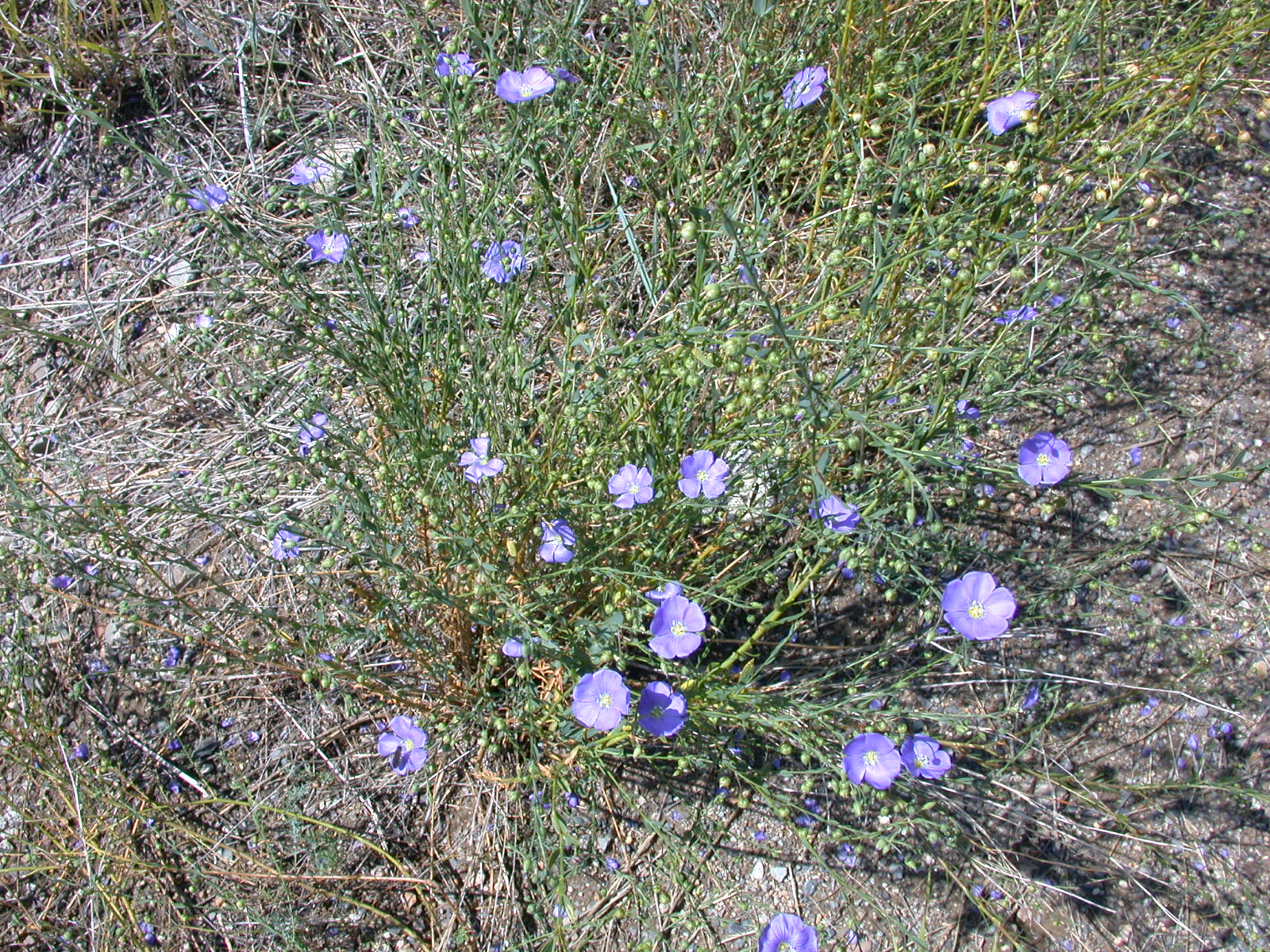The image captures a section of a barren, arid field on a sunny day, with a detailed close-up of a green plant bearing vibrant purple circular flowers, each with a yellow center and approximately the size of a quarter. The plant stands out in stark contrast to its dry surroundings, which consist of gray, black, and brown dirt, loose rocks, and scattered dead foliage and weeds. The flowers, radiating life amongst the desolate backdrop, have around five petals each. The ground beneath and around the plant appears cracked and parched, further emphasizing the harsh environment. The lighting suggests the photo was taken during the daytime, with prominent shadows stretching to the right, indicating the sun shining from the left.